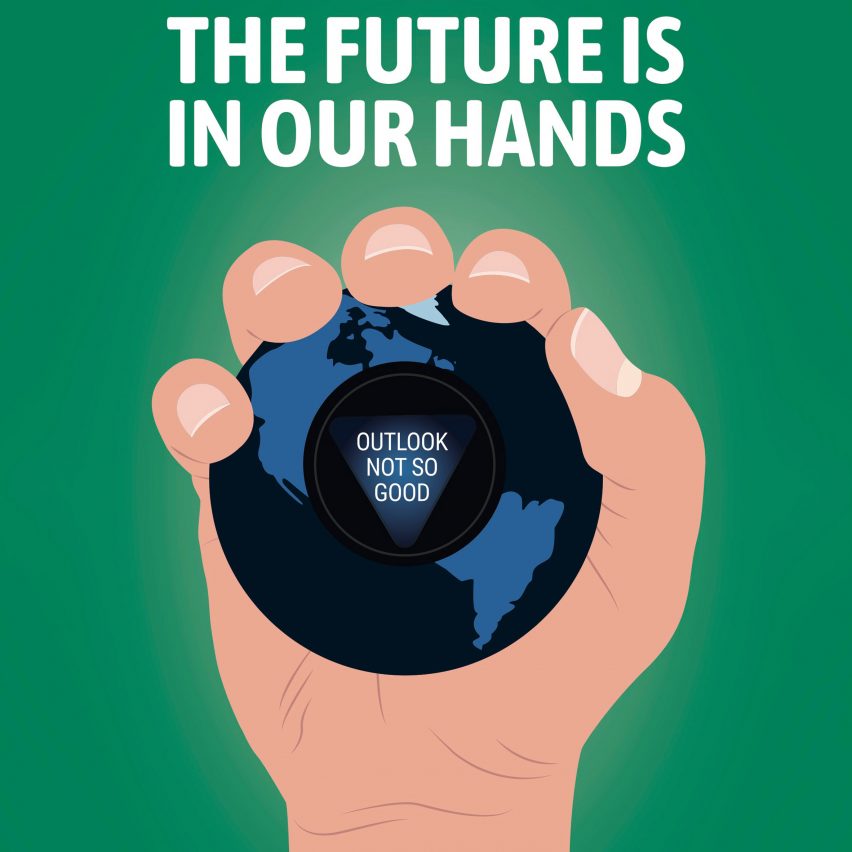This square, color digital illustration features a highly detailed drawing of an open right hand, centered against a green background. The hand, depicted with a light tan or beige skin tone, showcases its intricate details, including well-defined nails and palm lines. In the hand's grasp is a stylized Magic 8-Ball, which instead of its typical black color, features blue and dark gray patterning resembling a world map with identifiable continents like North and South America. Within the triangular window of the Magic 8-Ball, white text reads, "Outlook not so good." Above this central image, large white capital letters declare, "THE FUTURE IS IN OUR HANDS," making it clear this illustration is designed to convey a significant message, possibly for a poster or web design. Reflections on the Magic 8-Ball add a touch of realism to the otherwise illustrative work.